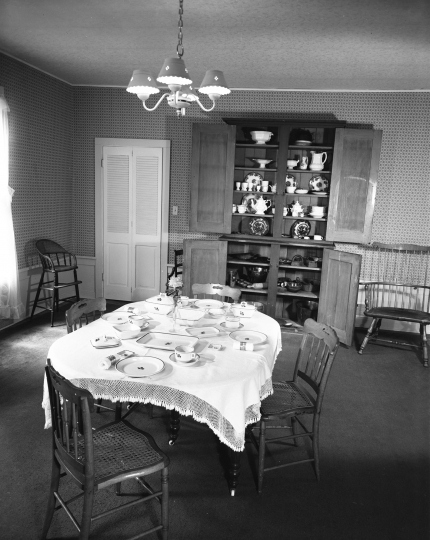This detailed black-and-white photograph, likely from the 1950s, captures the interior of a dining room. At the forefront of the image stands an oval-shaped wooden dining table, covered with a pristine white tablecloth. The table is set for four with white china, silverware, and various serving trays. Four wooden chairs, one on each side, surround the table. A flower vase, presumably the centerpiece, sits in the middle beneath a chandelier hanging from the ceiling.

To the left, light streams in through windows, just visible behind the edge of some curtains. The background features a large, open wooden China cabinet filled with an array of antique teapots, cups, and other kitchenware. Adjacent to the cabinet on the right is a solitary rocking chair. Two narrow doors on the left, suggestive of swinging doors, likely lead to the kitchen. The muted tones and scattered arrangement of objects evoke a nostalgic, yet cozy ambiance representative of mid-20th century domestic life.